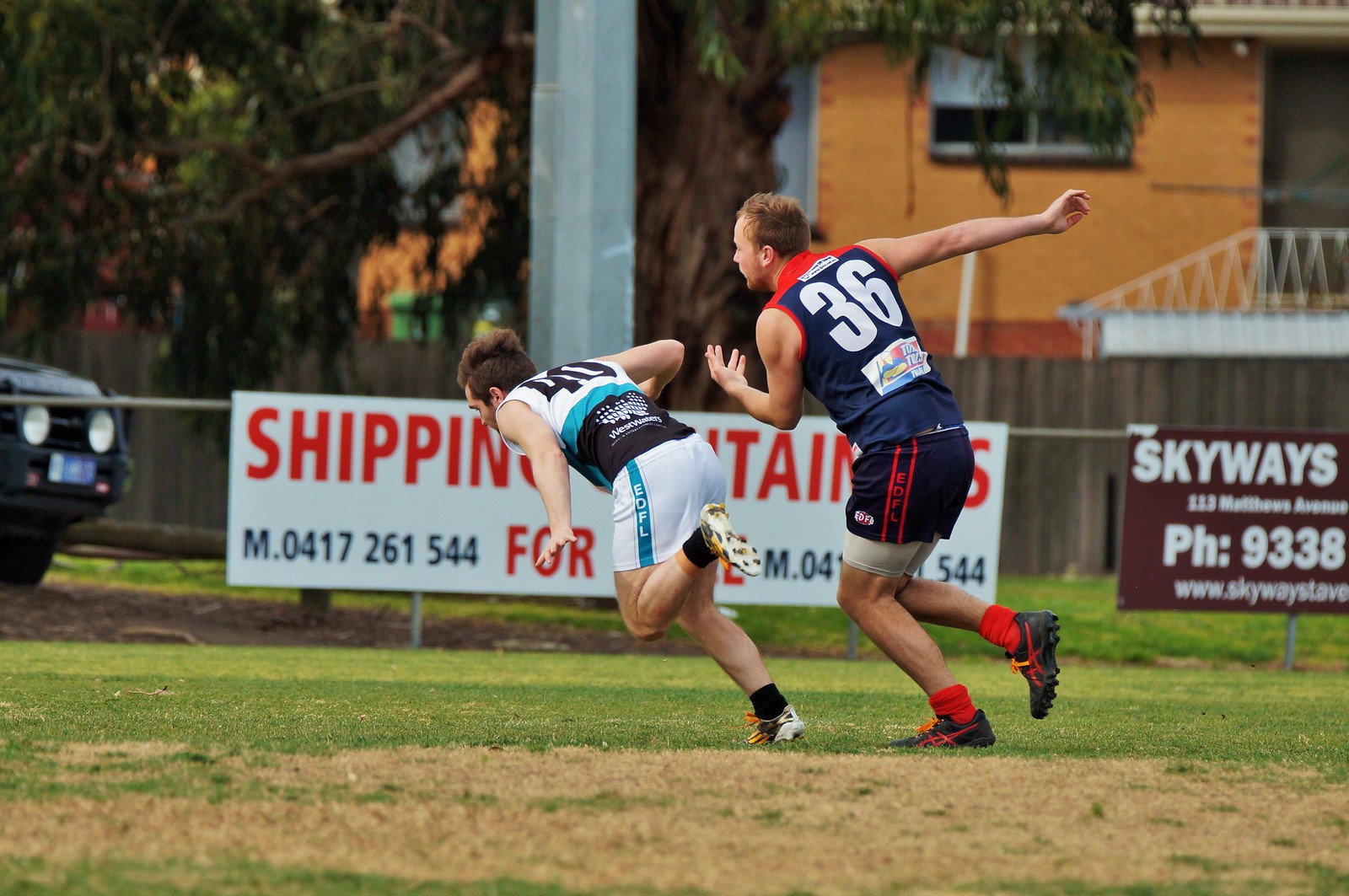In the center of the image, two athletes are captured in motion, running across a grassy lawn. The athlete in front, wearing a white jersey with the number 40 on his back, looks like he is about to trip as he leans precariously forward towards the left side of the image. He is dressed in a complete white outfit, including white shorts and sneakers, complemented by black socks. Trailing behind him on the right side is another athlete donning a navy blue jersey paired with navy blue shorts, red socks, and black sneakers, displaying the number 36 on his back.

The image is set outdoors, and the background features several elements. To the top right, a brown house stands out, along with a tree and a large pole. Part of the front of a car is also visible, adding to the suburban feel. There are multiple signs along the lawn; one reads "shipping" partially obscured by the runners, displaying the incomplete phone number M.0417261544 in red letters. Another sign, brown in color, bears the word "Skyways" and includes a phone number, though it is not fully visible. Some advertisement posters add further context, underscoring the setting's mix of residential and advertising elements.